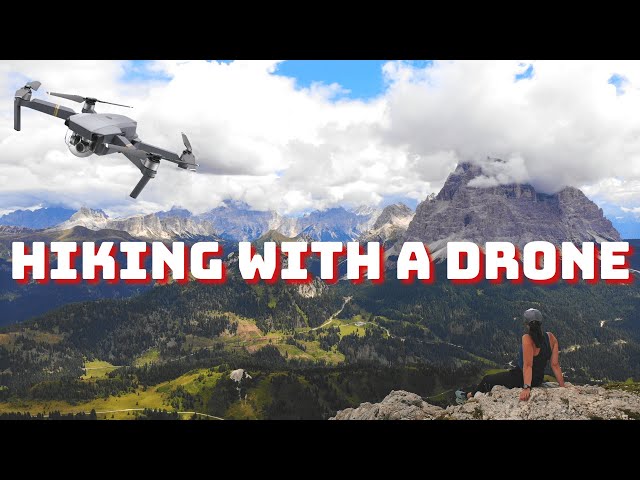The image showcases a breathtaking outdoor scene under a clear blue sky filled with puffy white clouds. A majestic mountain range stretches across the background, with some of the peaks disappearing into the clouds. In the upper left-hand corner, a gray drone hovers, ready to capture the natural beauty below. Bold white lettering, outlined in red, prominently reads "Hiking with a Drone" across the middle of the image, suggesting an adventurous theme. 

In the foreground, a female hiker with long dark hair sits atop a pile of rocks, wearing a black tank top, black pants, and a trucker-style ball cap. She gazes over a canyon lush with trees and verdant grass. A subtle black band outlines the bottom of the image, framing the scenic vista and enhancing the overall composition. This captivating scene elegantly combines elements of nature, adventure, and technology.